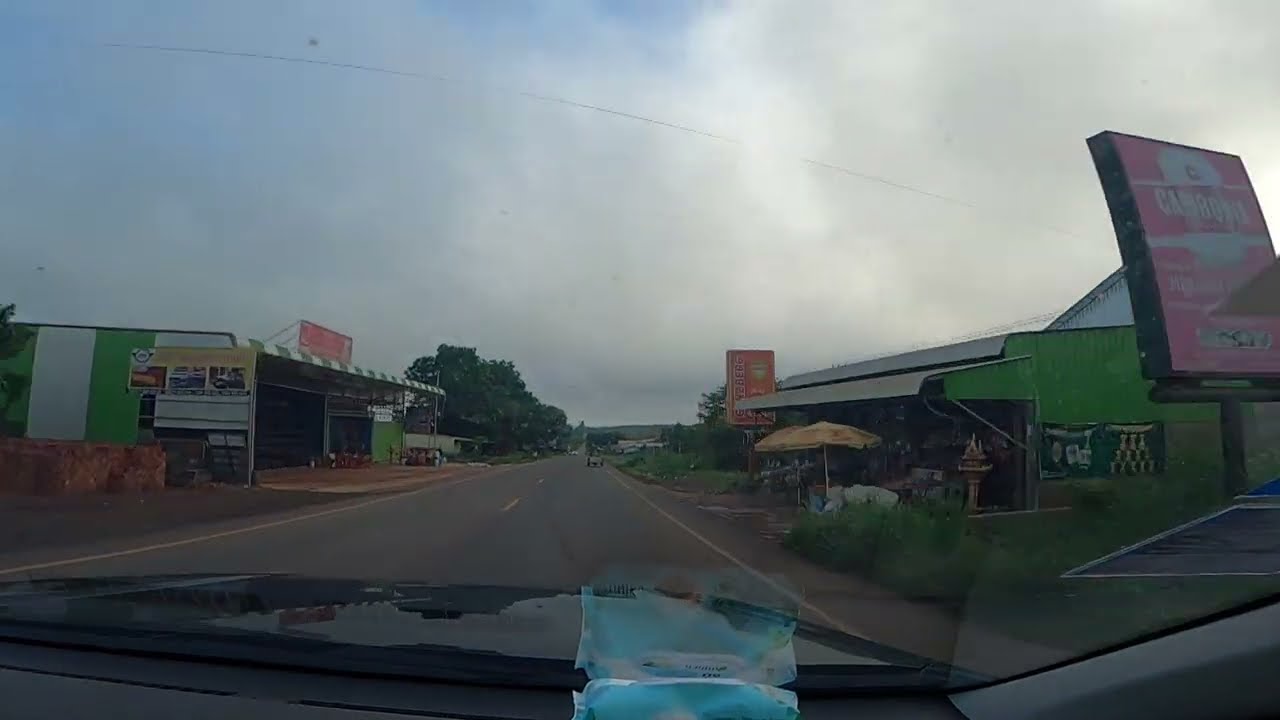The image captures a view through the windshield from the inside of a car traveling down a two-lane road in a small, seemingly underdeveloped town. Dark and gray clouds dominate the sky, with just a small patch of blue near the center. The dashboard of the car features a blurry blue object, potentially a bag of wipes or tissues, reflecting slightly on the windshield. To the right of the road, there's a one-story green building with yellow umbrellas pitched in front of it and an illegible red sign. On the left, another single-story building showcases green and white vertical stripes and a matching awning, accompanied by a banner that remains unreadable. The road is lined with dashed yellow lines in the center and white lines on the edges, and far down the road, another vehicle is visible. Trees can be seen in the distance on both sides of the street, adding to the serene, albeit overcast, rural setting.